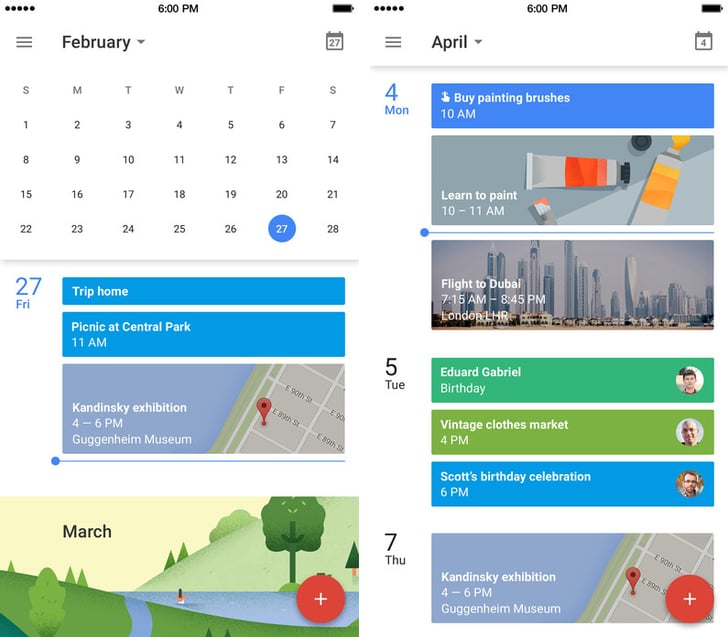The image showcases two side-by-side mock-up screenshots of a smartphone calendar app, arranged in a detailed and organized layout. The left screenshot displays a calendar for February, featuring various interface elements such as a hamburger menu, battery indicator, and a prominent “6pm” timestamp in the center. 

At the top, there are five small dots in the upper left corner, indicating notifications or other icons. The calendar grid shows the month of February, starting with Saturday the 1st and ending with Sunday the 28th. The current date, the 27th, is highlighted in blue. In the top left corner of the screen, it reads "27th and Friday."

Below the calendar grid, there are three event fields:
1. The first event is marked in blue and labeled "Trip Home."
2. The second blue-marked event is "Picnic at Central Park," scheduled for 11 am.
3. The third event, denoted by a light blue color, has a Google Maps icon and reads "Kandinsky Exhibition, 4-6 pm, Guggenheim Museum."

Beneath these events, there is an option labeled "March," followed by a scenic graphic depicting a field, a path, a lake, and trees. A red circular plus button is featured at the bottom right corner of the screen.

The right screenshot displays a similar layout but is set for April 4th, which is a Monday. The date “April 4th” is highlighted, along with the day's weather, and a series of scheduled events:
1. "Bluefield by Painting Brushes," scheduled for 10 am, is accompanied by a paintbrush icon.
2. "Learn to Paint," from 10-11 am, with an icon of paint tubes.
3. A travel event titled "Flight to Dubai," showing a flight from 7:15 am to 8:45 pm, departing from London LHR.

Below these events, for Tuesday the 5th, there are three event entries:
1. "Edward Gabriel Birthday," marked in light green.
2. "Finch's Clothes Market" at 4 pm, in a lighter green.
3. "Scott's Birthday Celebration" at 6 pm, in blue.

Each event contains a photo icon on the right. Another "Kandinsky Exhibition" event, identical to the one on the left screenshot, is scheduled for Thursday the 7th. The right screen also features a red circular plus button in the bottom right corner.